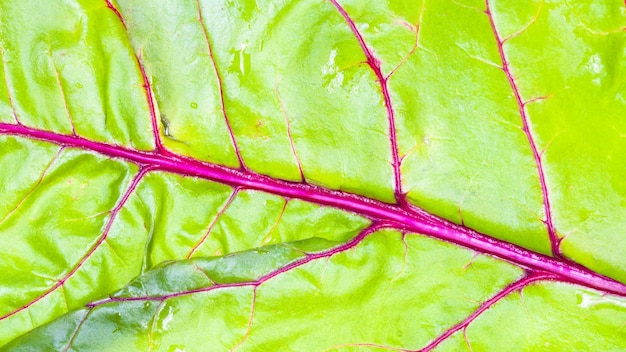This close-up photograph features a zoomed-in view of a leaf, possibly from a lettuce plant. The leaf displays a pale green to yellowish-green hue, appearing somewhat thin and rippled. The central vein is prominently thick and sports a bright, deep purple or slightly maroon coloration, while branching veins of varying thickness extend outwards from the center. These veins run at a slight tilt down to the right, and they have delicate, smaller branches that enhance the intricate veining pattern. The leaf itself appears waxy and supple, without any visible damage or blemishes. The background is entirely out of the frame, focusing solely on the detailed texture and color contrasts of the leaf. A light source in front of the leaf creates a subtle glare, highlighting its vivid colors and intricate structure.